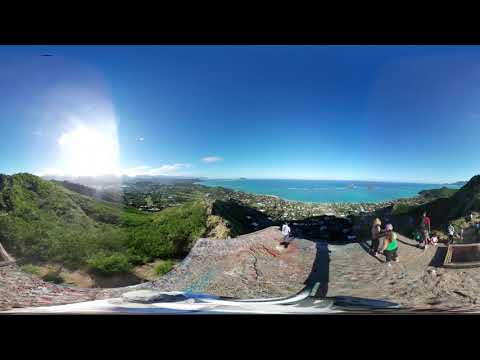This photograph showcases an expansive valley as seen from a gray, rocky cliff top overlook, where four people stand, some observing the panorama while others walk along a visible path on the right. The valley below is lush with greenery, teeming with grasses, trees, and rolling hills, gradually morphing into a cityscape with small houses nestled closer to the horizon. Beyond the city, a stunning expanse of bright teal sea stretches out, merging into a clear blue sky dotted with a few distant clouds. On the left side of the image, a bright white spot, likely the sun, can be seen peeking out along the horizon. The entire scene appears slightly curved due to a fisheye effect, with two horizontal black strips framing the top and bottom, adding to the unique visual presentation.